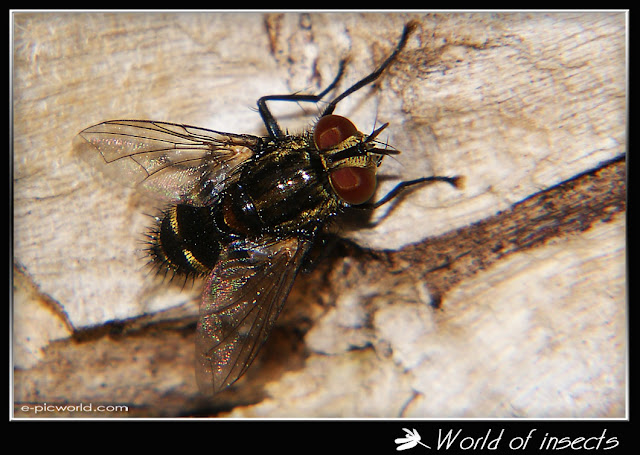This ultra close-up, colored photograph features a fly perched on a light brown wooden surface, possibly a table or tree bark. The image is surrounded by a black border with "world of insects" in white text in the lower right corner and "e-picworld.com" in the lower left corner. The fly's head is marked by striking red eyes and gold accents between them, complemented by small antennae. Its black body, adorned with thin, spiked hairs, shows two gold bands near the rounded bottom part. The transparent wings, edged with black, reveal the wooden surface beneath. Two prominent front legs and additional thin black legs on the sides enhance the close-up detail of the fly, all clearly visible due to the natural lighting of the scene.